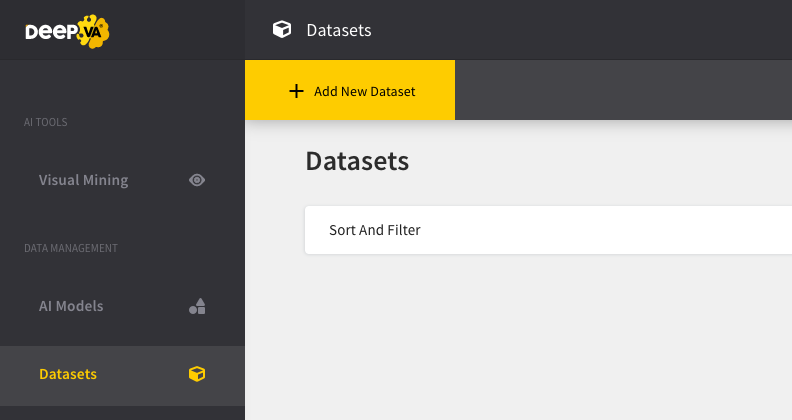The webpage for the Deep.va platform prominently features a dark gray color scheme encompassing the top and left sections. The website's name, "Deep.va," stands out with "Deep" in white letters, while ".va" is enclosed inside a yellow badge-like symbol with black lettering. Centered at the top of the page, "Datasets" is displayed along with a square icon to its left. Beneath this, a yellow rectangular box with a plus sign and the text "Add New Dataset" invites user interaction.

The main content area, set against a white background, begins with a bold "Datasets" header in black letters, followed by a filter box labeled "Sort and Filter." The dark gray left sidebar spans from top to bottom, starting with "AI Tools" at the top. Below this, "Visual Mining" is accompanied by an eye icon. Further down, "Data Management" precedes a section labeled "AI Models," each with its respective icons. At the very bottom of the sidebar, "Datasets" is highlighted in yellow letters with a small yellow box icon next to it.